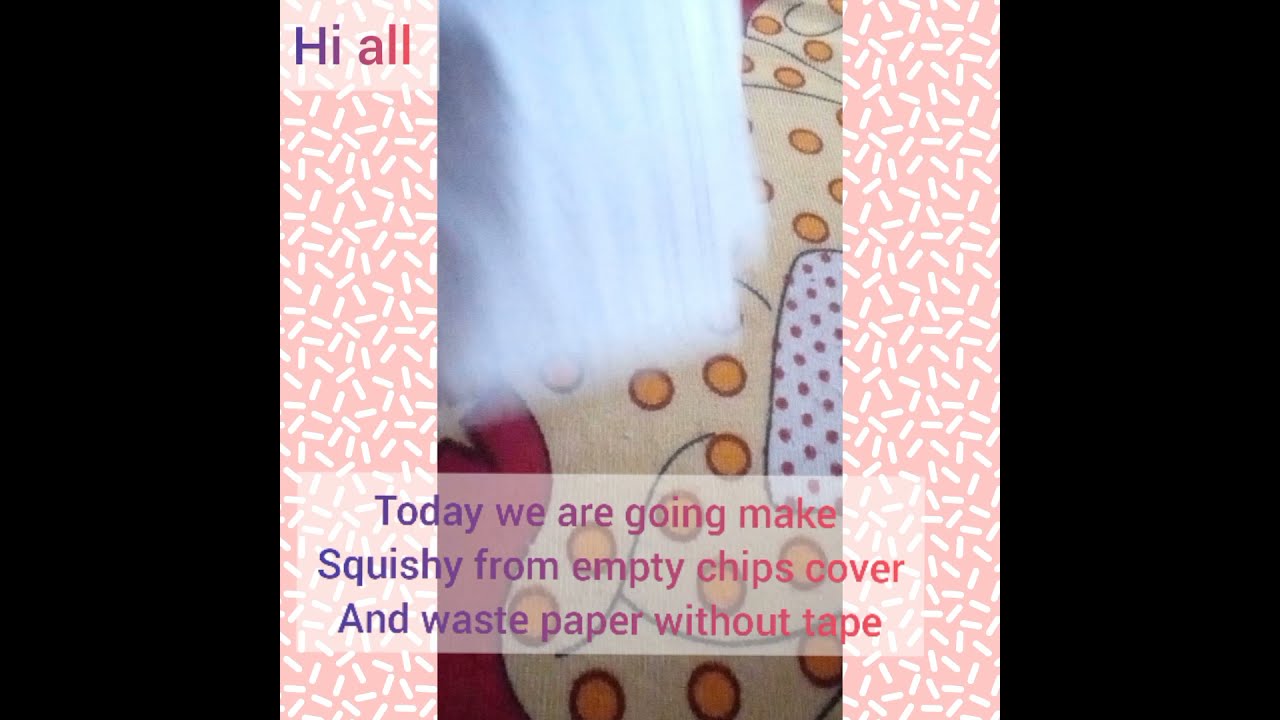The image is a vertically taken, digitally created collage. The background features a black screen, flanked by vertical pink stripes filled with white designs resembling sprinkles or rice. In the upper left corner, there is colorful text saying "Hi All." Below that, there is a central image that is partially blurry, showing some sheets of paper and a beige cartoon-like figure with little yellow circles and a polka-dotted white background. A red curvy object is also visible in the background. At the bottom of this central image, there is a slightly transparent white rectangle displaying the text: "Today we are going to make squishy from empty chips cover and waste paper without tape," divided into three lines. The text transitions in color from purple to a reddish-pink hue.